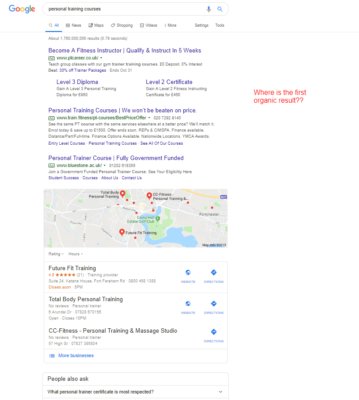This screenshot captures a Google search results page. The header displays the Google logo on the top left, despite the overall poor image quality. The search query entered is "personal training courses," as visible in the search bar. The "All" tab is highlighted in blue, indicating the current search category. Adjacent to the "All" tab are other options: "News," "Images," "Shopping," "Videos," and a "More" dropdown. Additionally, "Settings" and "Tools" buttons are positioned to the right.

The search results reveal no organic listings; each of the top three entries is marked with a green label indicating they are ads. This signifies that companies have paid for these placements to appear at the top of the search results. The far-right bottom corner shows red text highlighting a query about the first organic result, which points out the absence of such results on this page or screenshot.